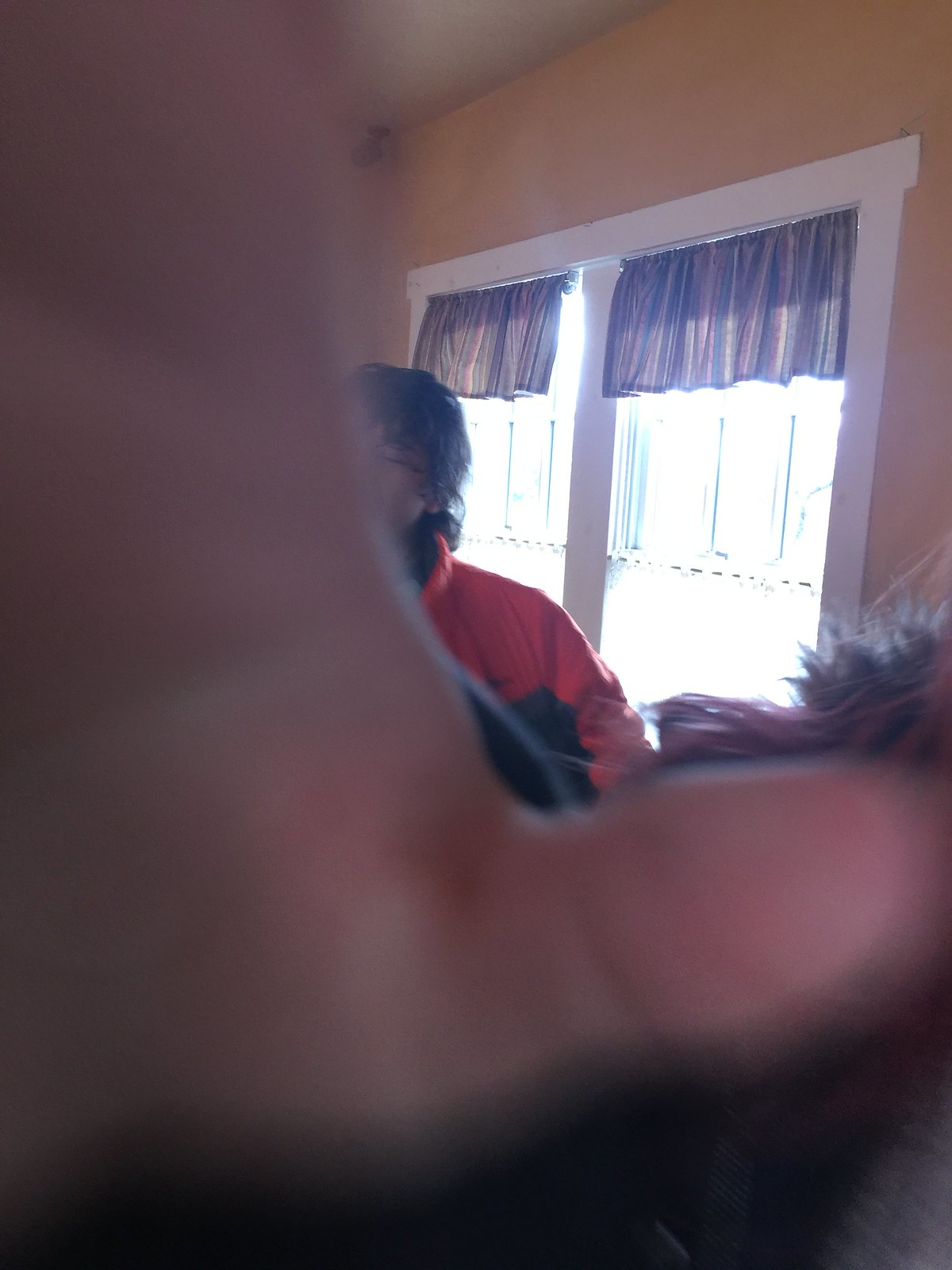A person's hand is prominently covering half of the camera lens, partially obscuring the view. In the background, there is an individual wearing a thin, red and black windbreaker jacket. Their medium-length hair drapes down, covering about half of their face, suggesting they are attempting to block the photograph with their hand. To the right, a double window allows a significant amount of sunlight to flood into the room. The window is adorned with small, dark-colored curtains at the top, which do little to diminish the brightness of the sunlight.